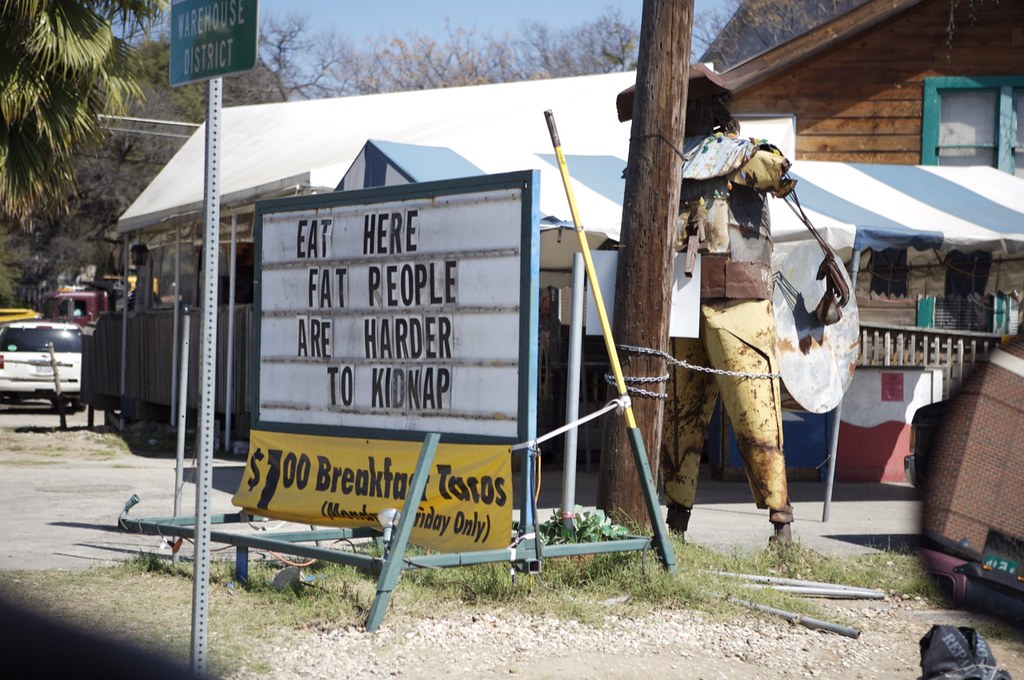In this vivid outdoor photograph taken under bright sunlight, the central focus is a marquee sign situated outside a restaurant. The sign, which is affixed to a green metal frame and positioned at eye level close to the ground, bears a humorous message in black letters on a white background: "Eat here, fat people are harder to kidnap." Below this, a yellow banner, possibly made of cloth or plastic, prominently advertises "$1 breakfast tacos" in large black letters.

In the backdrop, the base of a telephone pole is visible. Attached to this pole is a striking, scarecrow-like figure crafted from rusted metal, giving it an eerie, weathered appearance. This interesting decor element adds a unique character to the setting.

The restaurant itself, seen just behind the sign and the telephone pole, is a rustic wood-paneled building. The windows are framed in a distinctive teal color, adding a pop of color to the otherwise earthy tones of the structure. In the distance to the left, there are parked cars, suggesting that this might be a bustling tourist area. The overall scene evokes a quirky, inviting atmosphere that beckons passersby to stop and enjoy the local fare.